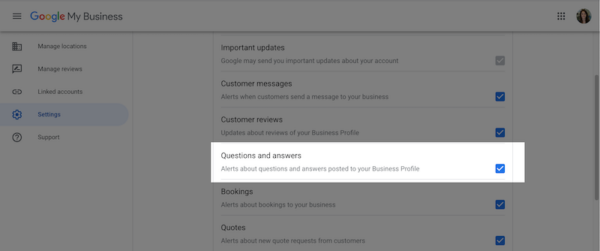The image is a landscape-oriented screenshot of a website, specifically of the Google My Business application. The majority of the screen has a gray overlay, with a central section highlighted in white, drawing attention to it. At the top left corner of the interface, there are three horizontal lines serving as a menu icon, followed by the title "Google My Business."

Along the left side of the screen is a vertical column with tab names listed in succession: "Manage Locations," "Manage Reviews," "Linked Accounts," "Settings" (this tab is highlighted in blue, indicating it is currently selected), and "Support." 

In the middle section of the screen, there is a list of options: "Important Updates," "Customer Messages," "Customer Reviews," "Questions and Answers" (this option is highlighted in white, signifying it is currently focused on), "Bookings," and "Quotes." Each of these options has a succinct description underneath it, and to their right, there are checkboxes. All options, except for "Important Updates," are checked in blue, indicating they have been selected.

Finally, in the top right corner of the screenshot, there is a small profile picture thumbnail, adding a personalized touch to the interface.